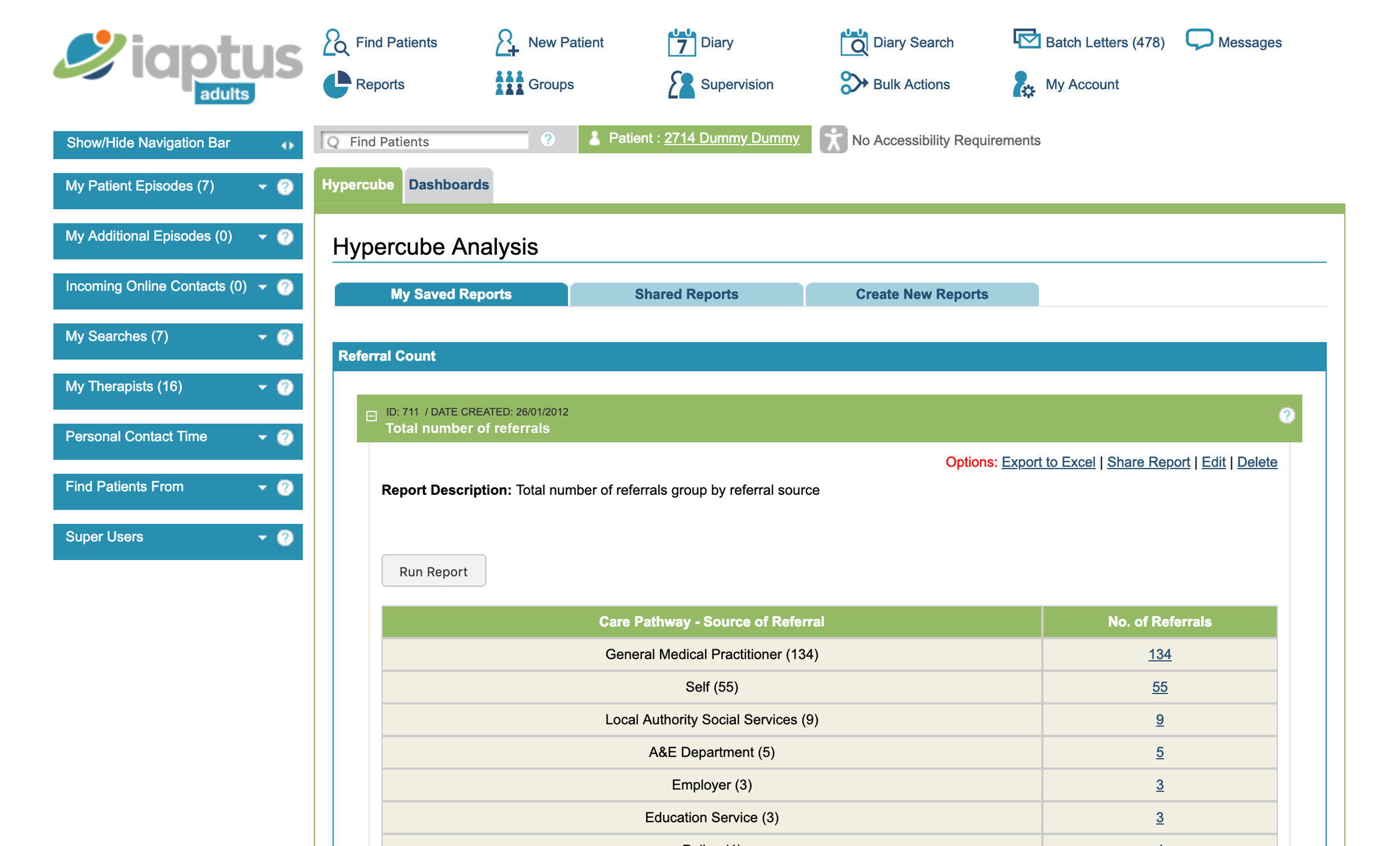The image depicts a website interface, featuring a main design element at the top—a planet illustration with a small orange circle situated on the planet's top-right. Surrounding the planet is a green ring. Below this graphic, the website's name, "iaptus," is displayed in lowercase gray letters.

Directly under the website's name, there is a small, blue background segment with "adults" written in white text. Spanning horizontally, the menu is organized into two rows. The first row includes options: "Find Patients," "New Patient," "Diary," "Diary Search," "Batch Letters," and "Messages." The second row consists of: "Search Reports," "Groups," "Supervision," "Bulk Actions," and "My Account."

Beneath the horizontal menu lies a gray search bar featuring a white input field labeled "Find Patients." An entry below this search bar reads "Patient 2714 Dummy Dummy," against a white background with the note "No accessibility requirements."

On the left side of the interface is a vertical menu with various dropdown options including "Show/Hide Navigation Bar," "My Patient Episodes," "My Additional Episodes," "Incoming Online Contacts," "My Searches," "My Therapists," "Personal Contact Time," "Find Patients From," and "Super Users."

On the same left-side menu, there is a section labeled "Hypercube Dashboards" which expands to "Hypercube Analysis," "My Saved Reports," "Shared Reports," and "Create New Reports." The interface also features report descriptors such as "Referral Count," "Total Number of Referrals," "Report Description," and "Total Number of Referrals, Grouped by Referral Source," with a note specifying "For any poor."